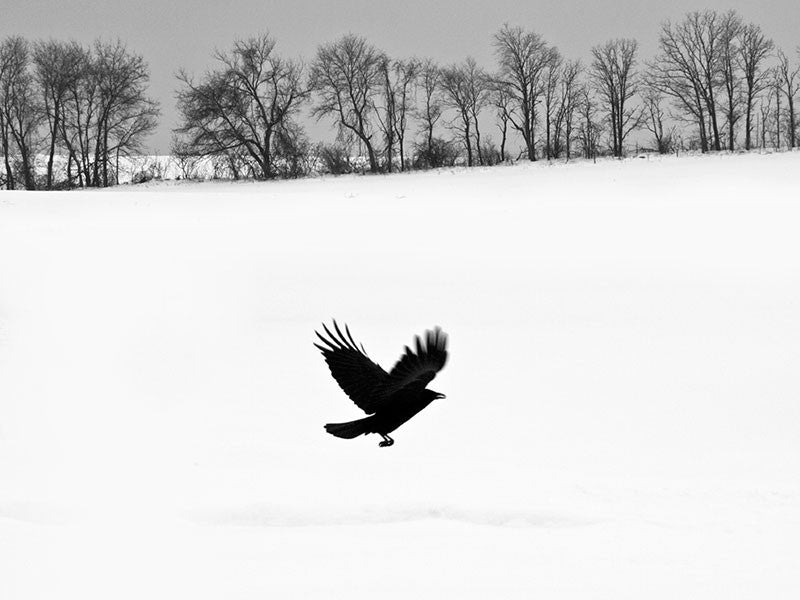In this black and white photograph, a black crow is captured in mid-flight over a pure white snowy field. The crow, centrally positioned near the bottom, has its wings outspread, with the feathers at the tips separated, and its beak facing the right side of the image. Its legs are curled up, and its tail points backward. The background features a row of bare, leafless trees, their dark silhouettes stark against the gray sky. Further in the distance, another field of snow stretches out, bordered by more trees on the horizon. The composition vividly contrasts the dark figure of the crow and the skeletal structure of the trees with the expansive, wintry landscape.